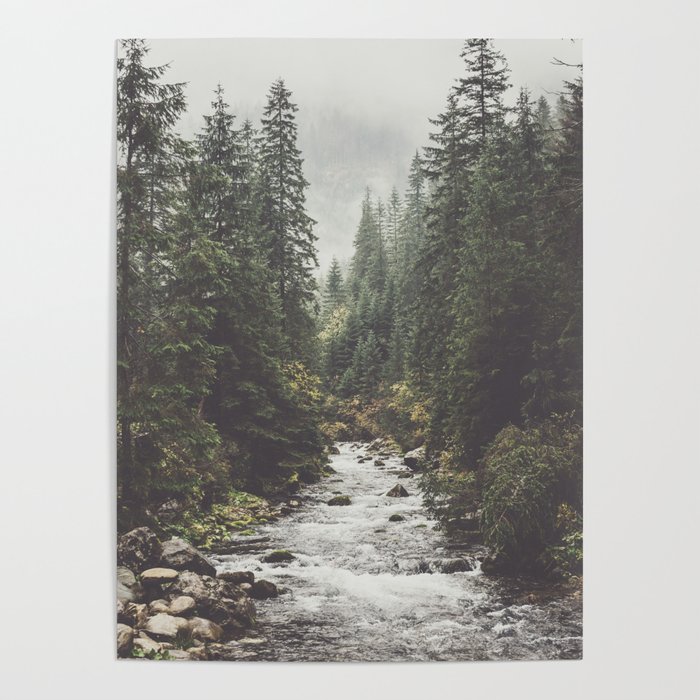The photograph, presented as a promotional image for an online shop, displays a vertically aligned, rectangular poster that appears to be lying on a flat light gray surface. The poster itself showcases a realistic photograph of a narrow, rough-looking river with white-tipped waves and several rocks sticking out from the shallow water. The river flows from the center toward the bottom of the image, flanked by shorelines covered in various vegetation, including tall green palm and conifer trees. The lush forest on either side contrasts with the rocky riverbed, and some of the trees lean noticeably, with one prominent conifer appearing to be tipped forward. Additionally, the upper portion of the photograph shows a gray, cloudy sky with darker areas in the center and lighter gray along the top. In the far distance, fog and mist shroud the landscape, with mountains or hills subtly rising in the background, adding depth to the scene.